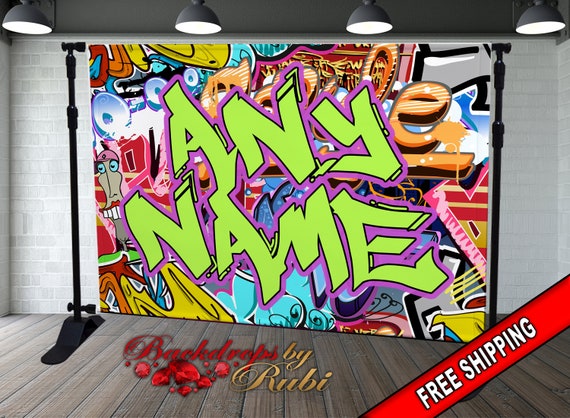This image is a detailed advertisement for customizable photo backdrops, resembling a vibrant piece of graffiti art. The backdrop is displayed on a sturdy plastic black pipe stand, featuring two vertical poles with a flared base and a horizontal connecting pole at the top. This structure is set against a wood floor with a neutral white brick background and hanging studio lights above.

The backdrop itself is a strikingly colorful cartoon graffiti, showcasing overlapping three-dimensional letters and stylized faces in hues of light blue, orange, yellow, red, green, and purple, creating a dynamic 80s vibe. Dominating the center of the backdrop, large green letters outlined in purple spell out "any name" in a slanted graffiti style, emphasizing the customizable nature of the product.

In the lower right corner, a diagonal red ribbon displays the bold text "Free Shipping" in white. Additionally, at the bottom of the backdrop, there's a logo that reads "Backdrop by R-U-B-I," adorned with raw ruby gem illustrations, marking the brand's signature style. This image overall conveys the vibrant, customizable, and promotional features of the photo backdrop effectively.